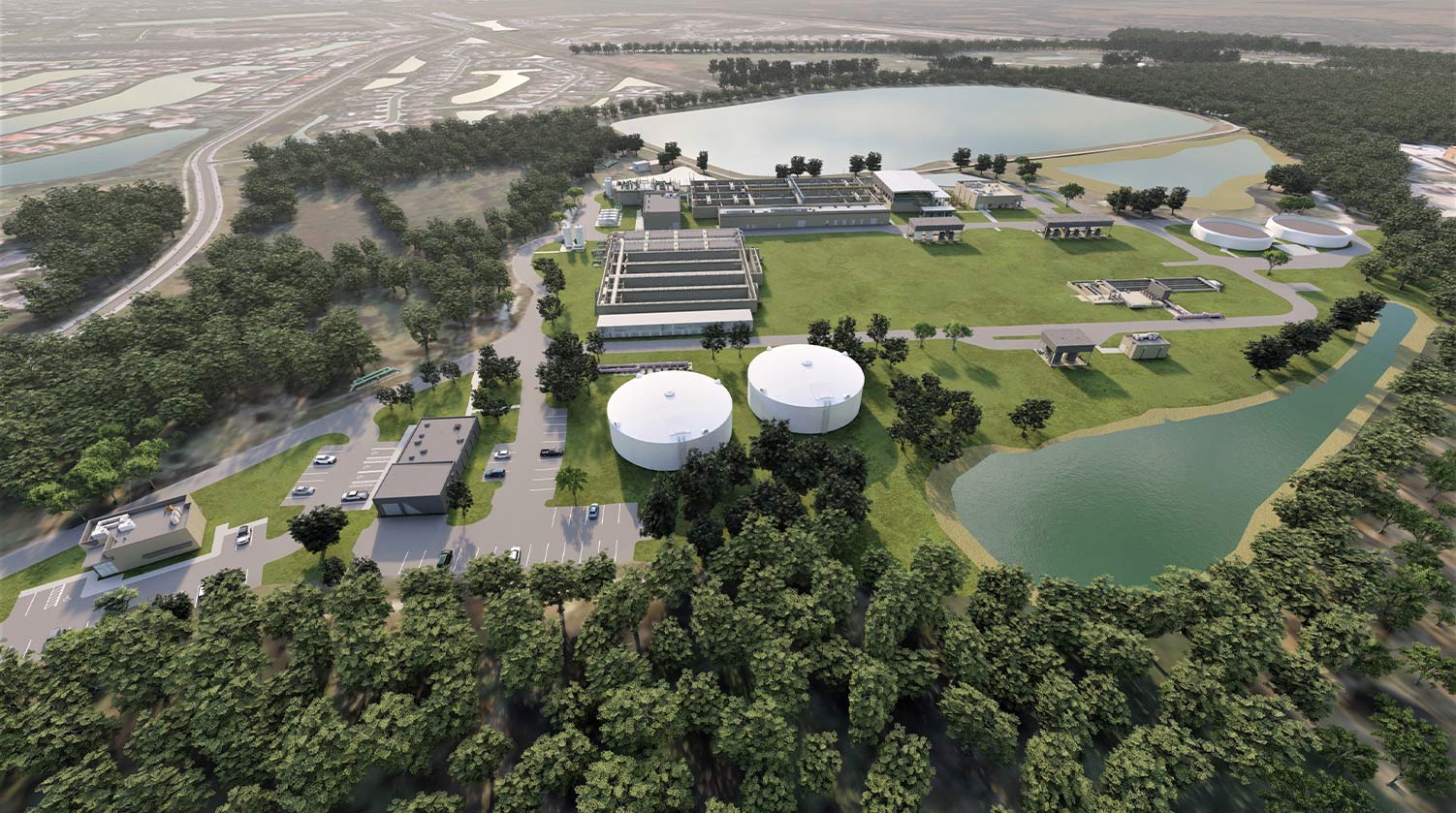This bird's eye view image captures a detailed landscape dominated by a water treatment facility, characterized by two prominent white circular structures that resemble large containers or domes, centrally located. These are flanked by lush green trees that extend across the entire bottom and right side of the image, providing a verdant contrast to the industrial elements. Adjacent to these domes, there are additional treatment areas, including two open sections situated at the back right, likely serving specific functions within the facility. To the immediate left, various rectangular buildings can be seen, with tan and gray rooftops, complemented by a reception office and a small adjacent building on the lower left side. The image also highlights several gray roads weaving through the area, parking lots peppered with white, silver, black, and blue cars, and delineated by white parking lines. Towards the top, the land transitions into flat terrain interspersed with bodies of water; to the left is a greenish water body framed by trees, while other segments contain more grayish waters. A foggy backdrop enhances the depth, encompassing more green trees and blurring into the horizon, where additional gray structures and land-water intersections are visible.